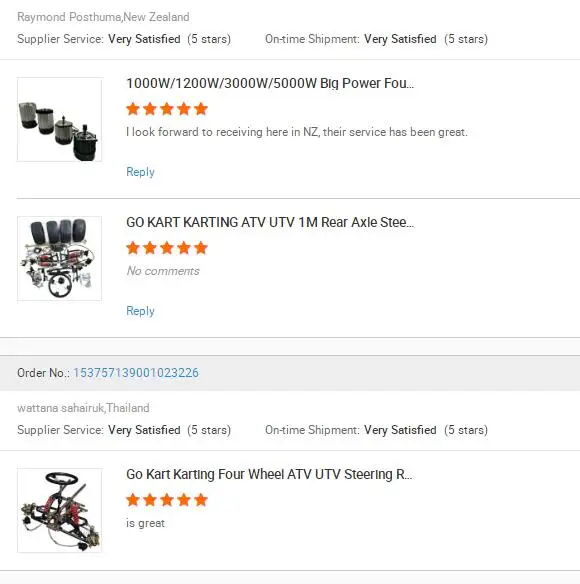The image depicts a series of customer reviews for various products from different suppliers. The first review is from Raymond Postma in New Zealand, who praises the supplier for their excellent service, awarding five stars for both supplier service and on-time shipment. He is particularly satisfied with a range of high-power products, including 1,000-watt, 1,200-watt, 3,000-watt, and 5,000-watt equipment, and mentions that he eagerly awaits their arrival in New Zealand.

Another review is from Watana Saruk in Thailand, who also rates the supplier service and on-time shipment with five stars each. This review pertains to a go-karting, ATV, UTV, 1M rear axle made of steel. Saruk did not leave additional comments but expressed high satisfaction through the five-star ratings.

The image includes visual references to parts such as a pole with a wheel on top, a steering wheel, some additional wheels at the bottom, wires, and what appear to be air filters. Each component is linked to the high satisfaction ratings provided by these customers, highlighting the quality and reliability of the supplier services.